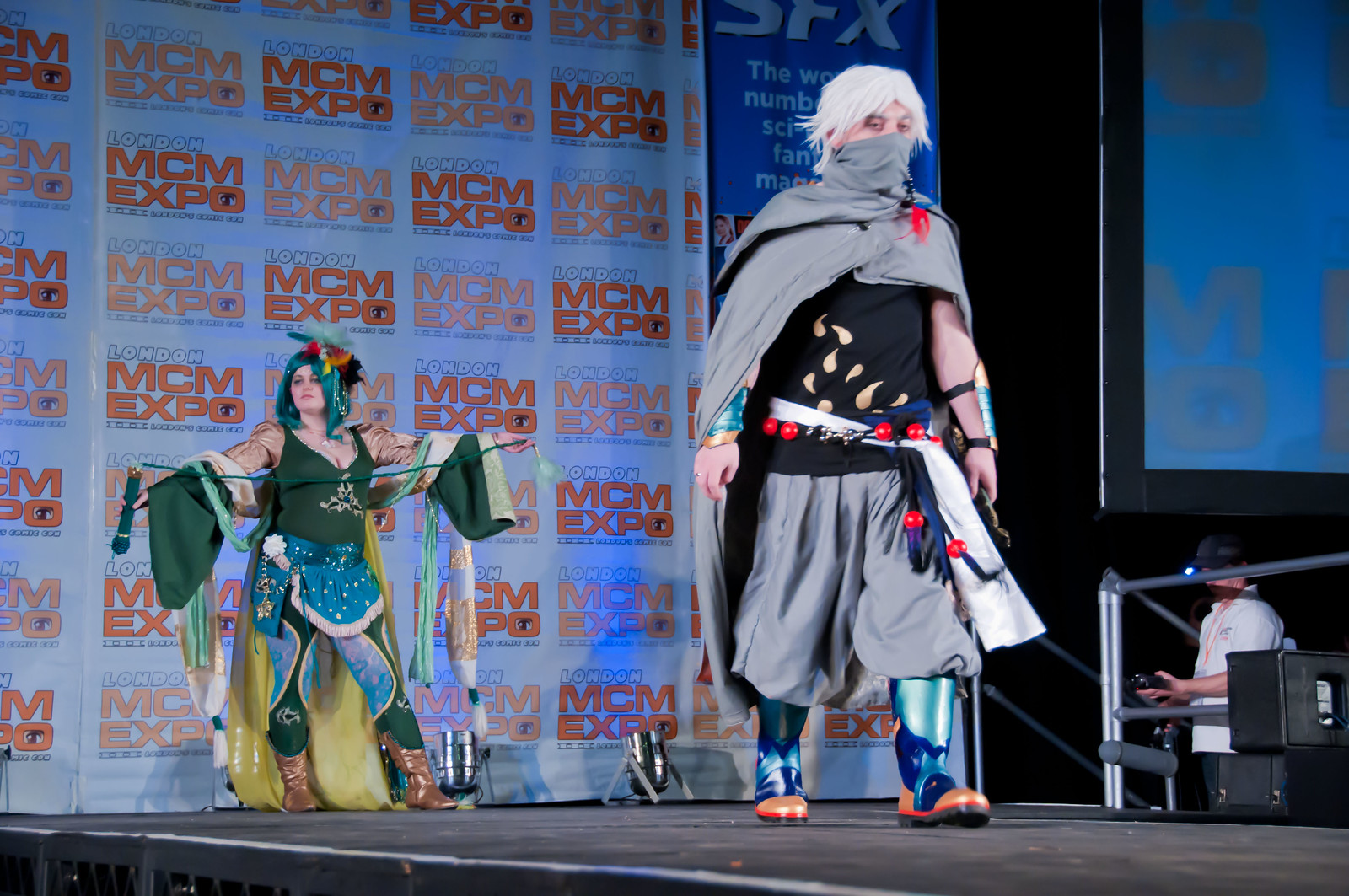The image showcases an indoor color photograph of a stage at the London MCM Expo, where two elaborately costumed individuals are featured. In the foreground, a person with white hair, partially obscured by a gray hood or cloak that covers the lower half of their face, walks towards the camera. They are donned in a black shirt adorned with light brown teardrop designs, blue and gold arm bracers, a sash with gray and blue material and red spheres, baggy gray pants, and colorful plastic boots with orange toes and light teal accents up the ankles. 

Further back on the stage, a woman stands with arms outstretched, holding a green object in one hand and a rope in the other. She sports a green wig or elaborate hairpiece, a green tank top, a blue skirt, green and blue leggings, and brown boots. The backdrop features a repeating white logo that reads "London MCM Expo," arranged in a grid of squares. To the right, a man in a white shirt and black cap can be seen engaged in backstage work, in front of a large digital screen.